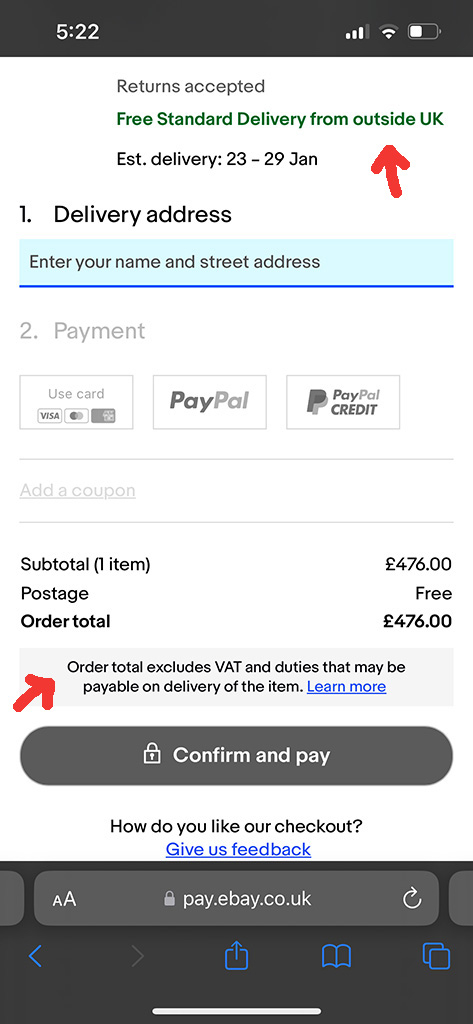The image depicts a vertical rectangular section of what appears to be a cell phone screen with an online checkout interface. 

### Header:
- At the very top is a black horizontal rectangle displaying the time "5:22" in white font on the left. On the right, various icons including a half-filled battery indicator are displayed.

### Main Content:
- **Title**: Below the header, slightly left of center, "Returns Accepted" is written in black font.
- **Delivery Information**:
  - In green font, it reads "Free standard delivery from outside UK." A red, hand-drawn-looking arrow points to the word "outside."
  - In black font, "Est. delivery: 23-29 Jan."

### Sections:
1. **Delivery Address**:
   - The label "1. Delivery Address" is in black font.
   - A light blue input field is underneath, prompting users to "Enter your name and street address," with a bright blue underline highlighting the field.
2. **Payment Method**:
   - "2. Payment" is grayed out but visible, along with three horizontal rectangles representing different payment options:
     - "Use Card" with icons for Visa, MasterCard, and another payment card.
     - "PayPal"
     - "PayPal Credit"
   - "Add a Coupon" is also grayed out beneath these options.

### Order Summary:
- **Cost Breakdown**:
  - In black bold font, "Subtotal (1 item): £476.00"
  - To the left, "Postage" is listed, with "Free" to the right.
  - "Order Total" is listed on the left, with "£476.00" on the right.
- In a gray shaded area, a note in black font states, "Order total excludes VAT and duties that may be payable on delivery of the item." 
  - "Learn More" is underlined in blue, with a red arrow pointing to the word "Order."

### Final Steps:
- **Confirmation**:
  - A dark charcoal gray oval button reads "Confirm and Pay" in white font, accompanied by a small logo on the left.
- **Feedback**:
  - Below the button, "How do you like our checkout?" is asked in black font. 
  - "Give us feedback" is underlined in blue on a white background.
- **Footer**:
  - At the bottom, another black rectangular area includes a charcoal gray horizontal oval with a web address written inside and some phone icons at the bottom.

The detailed layout of the checkout interface provides a clear and comprehensive description of the online shopping process, with emphasis on user interaction points and necessary information.